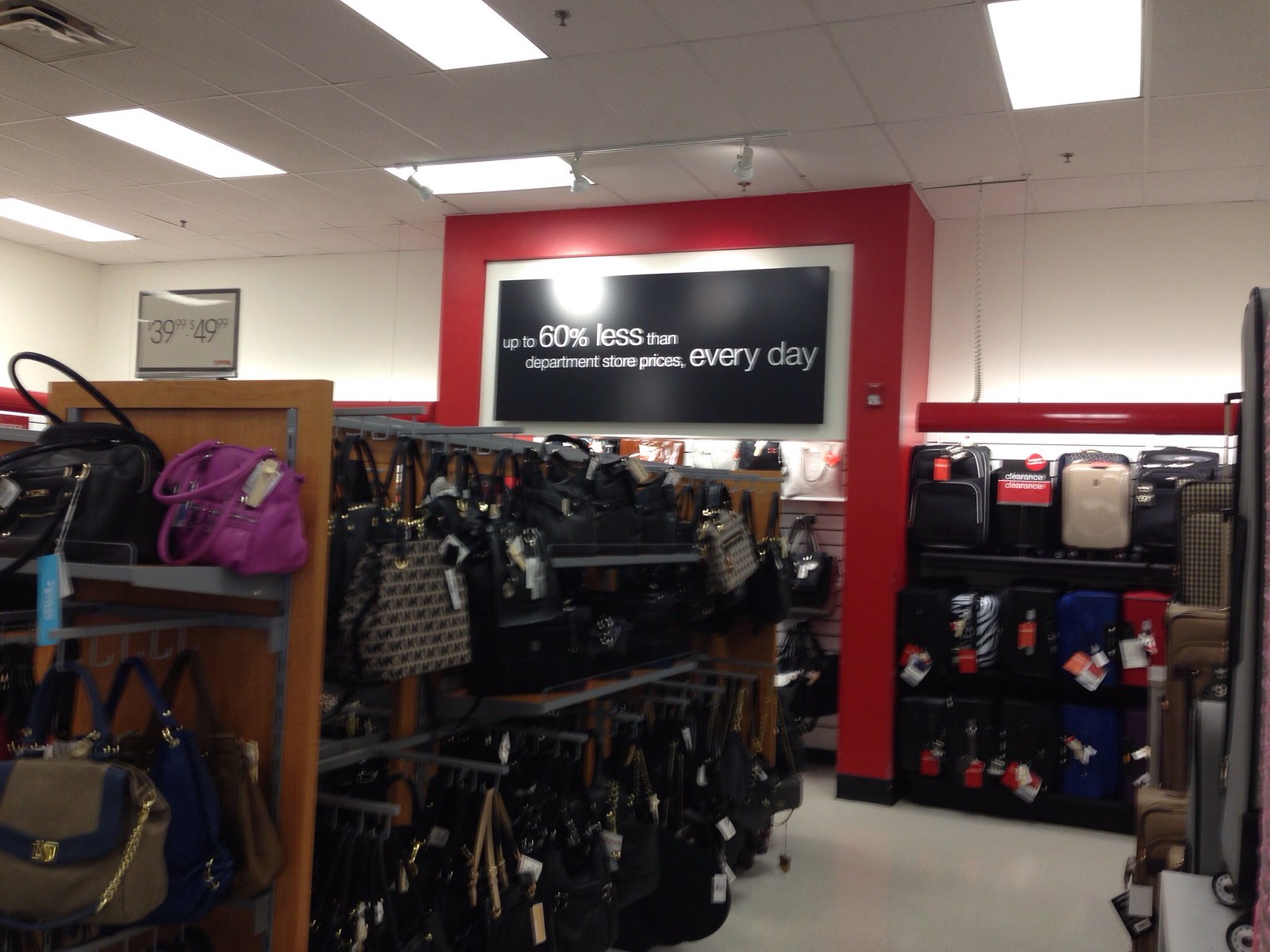This image captures the interior of a retail baggage store, possibly a discount outlet such as Ross or Burlington. Dominating the top portion is a white drop ceiling featuring two visibly installed lights on the left and another further aligned towards the center. Beneath this ceiling, a prominent red horizontal beam spans across the store, bearing a large black sign bordered in gold or silver, which reads, "Up to 60% less than department store prices every day." Adjacent to this beam, the back wall is painted white with several red accents extending to the right edge of the frame.

Below this signage, several shelving units display an array of luggage options. Three main shelves hold various suitcases arranged against the wall. In front, a prominent wooden display system features numerous hooks and shelving that showcase around 100 purses, ranging from small clutches to larger shoulder and tote bags. These displays are richly populated, especially on the left side where black and brightly colored purses are densely packed.

Further down, towards the left, additional shelves display pricing signage marked at $39.99 to $49.99. The grey flooring before the display provides a contrasting backdrop. More luggage is stacked halfway up the right side of the image, providing a comprehensive view of the store's diverse baggage options, including carry-ons and larger suitcases.